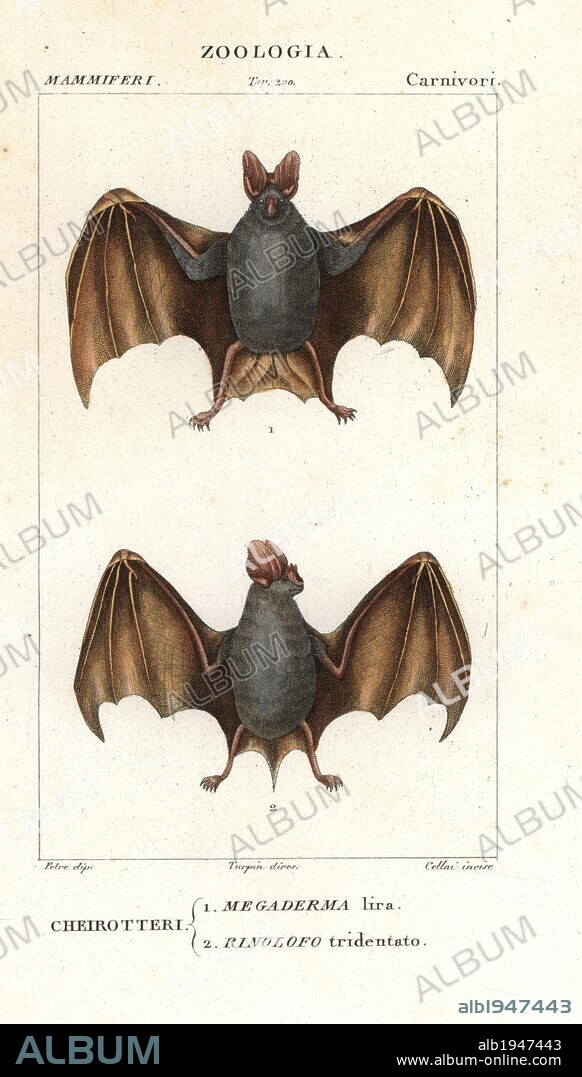The image is an informational card about a bat, set against a tannish white background. At the very top, the card features black text that reads "Zoologia, Mammiferi, Carnivori." Central to the card are two detailed drawings of the same bat. The first drawing shows the bat with a gray body, brown wings, and brown legs, arms, and ears, facing forward. The second image depicts the same bat with its head turned to the right, emphasizing its ears. Below the images, in a more detailed section, it reads "Chirotteri Megaderma lyra of Binolopha tridentato." At the bottom of the card, a black border displays the text "Album ALB1947443" and a web address, "www.album.online.com." The color palette includes shades of black, gray, brown, and beige. Additionally, a watermark with the text "album" is slanted and repeated throughout the image, giving it the appearance of a magazine or flyer.